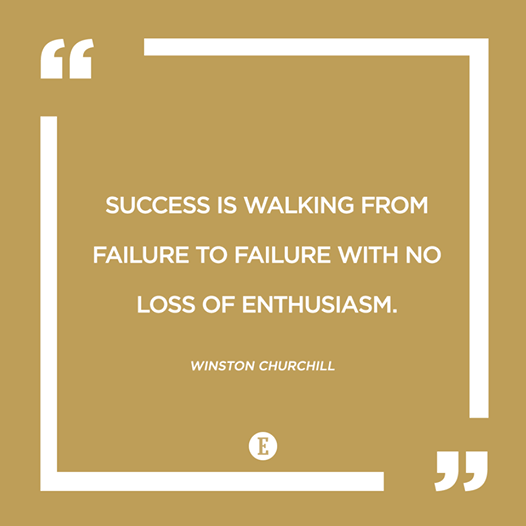The image features a gold or beige background with a clean, minimalist design intended as a motivational quote. At the top left and bottom right corners, white quotation marks frame the quote, while white L-shaped (or right-angle) borders adorn the top right and bottom left corners, adding structure to the composition. In the center, the quote is displayed in large, capitalized white letters, stating: "Success is walking from failure to failure with no loss of enthusiasm." Beneath the quote, in smaller letters, is the attribution to Winston Churchill. At the very bottom of the image, there is a white circle containing a white letter "E" in the same gold or beige color as the background, acting as a simple logo. Overall, the image conveys a polished and motivational aesthetic, suitable for framing and displaying in an office or personal workspace.